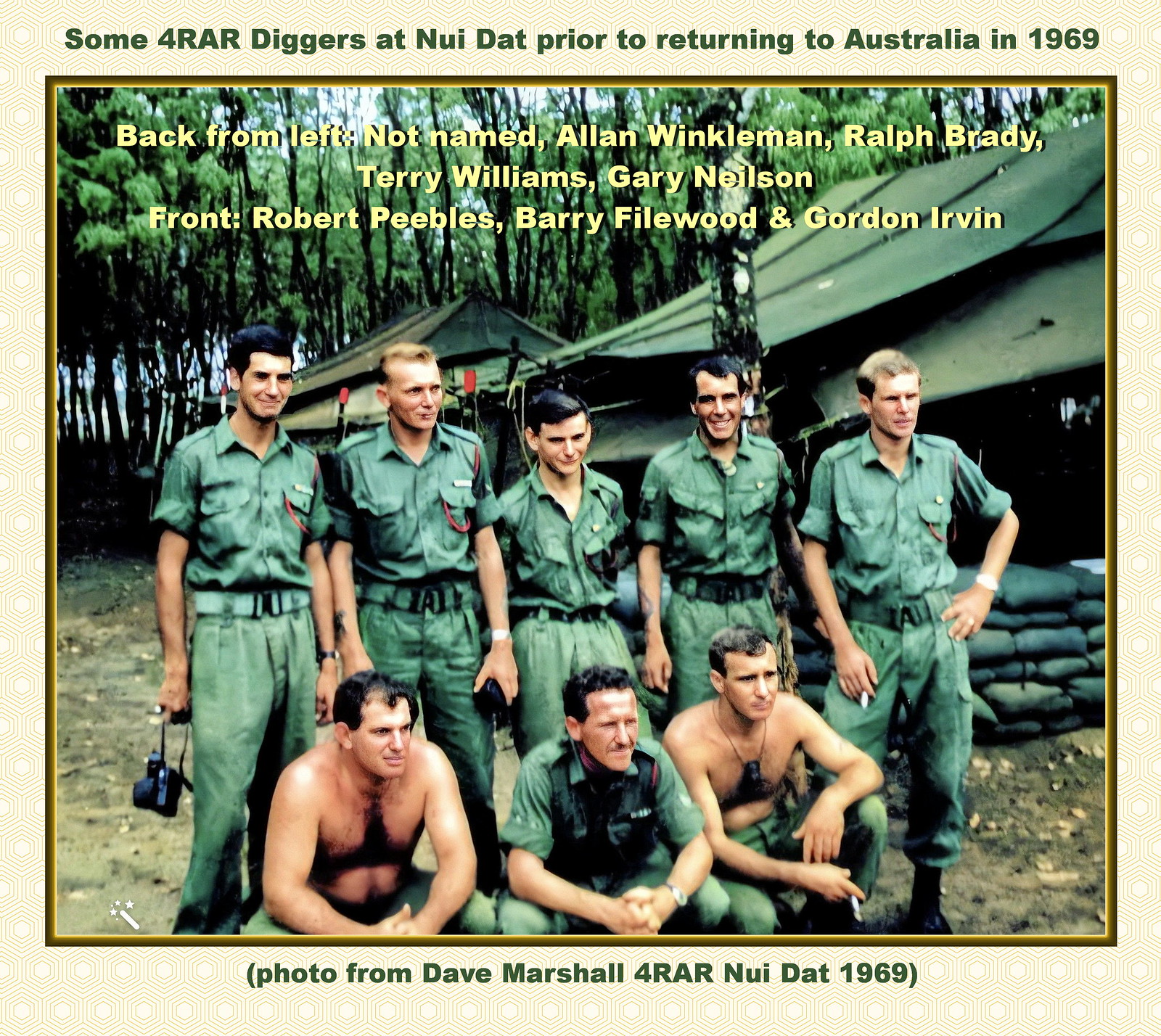The image features a vintage photograph of a military troop, specifically a group of soldiers from the 4th Battalion, Royal Australian Regiment (4 RAR), posing in front of their camp at Nui Dat prior to their return to Australia in 1969. The troops are situated in a forested area with visible army tents and sandbags in the background. The green text at the top of the image reads, "Some 4 RAR diggers at Nui Dat prior to returning to Australia in 1969." Below this, yellow text lists their names from left to right. 

In the back row, five men are standing:
1. Alan Winkerman 
2. Ralph Brady 
3. Terry Williams 
4. Gary Nielsen 
5. An unnamed individual 

In the front row, three men are crouched down:
1. Robert Peoples, on the left, who is shirtless, with black hair and a stern yet grinning expression
2. Barry Filewood, at the center, wearing a shirt and a watch on his left wrist, with a serious demeanor and a prominent forehead
3. Gordon Irving, on the right, also shirtless, brown-haired, smoking a cigarette, with dog tags and green army pants

The bottom of the photo notes, "Photo from Dave Marshall, 4 RAR, Nui Dat, 1969," emphasizing the historical context of the image. The soldiers, mostly dressed in standard-issue green army shirts and pants, exude a youthful appearance, highlighting the era and circumstances of their service.